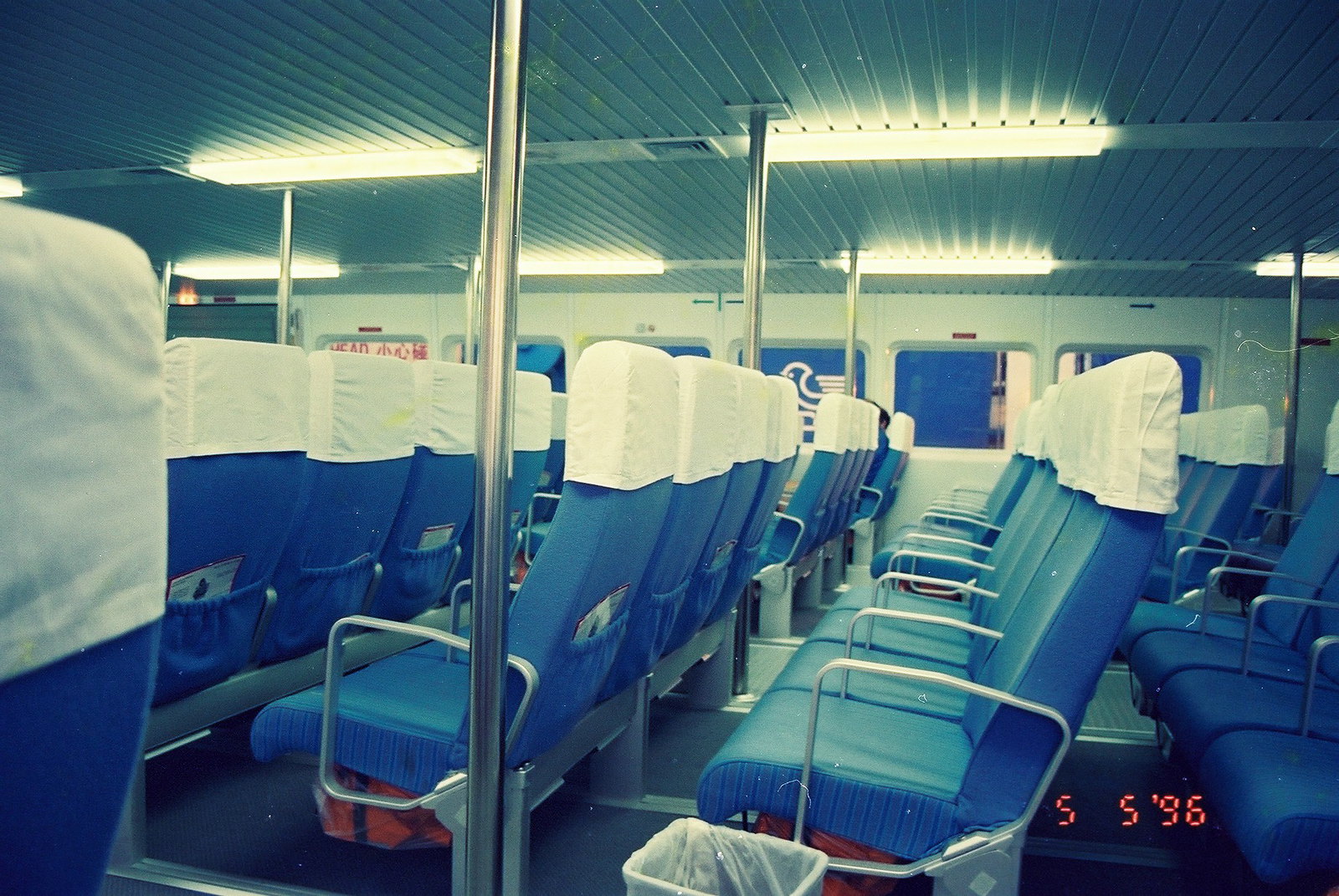This photograph captures the interior of a large transport vehicle, possibly a train or a ferry, dated 5-5-96. The image provides a side view of four rows of blue seats, each adorned with a white covering at the headrest designed for easy replacement. In the foreground, a wastebasket is positioned at the beginning of one row of seats. Underneath many, but not all, of the seats, there are orangish bags partially visible. The cabin features several silver poles running from the floor to the ceiling, providing structural support. The ceiling itself has inset white lights, contributing to the overall illumination. The floor appears to be covered in a black carpet, adding a sense of cohesion to the interior decor.